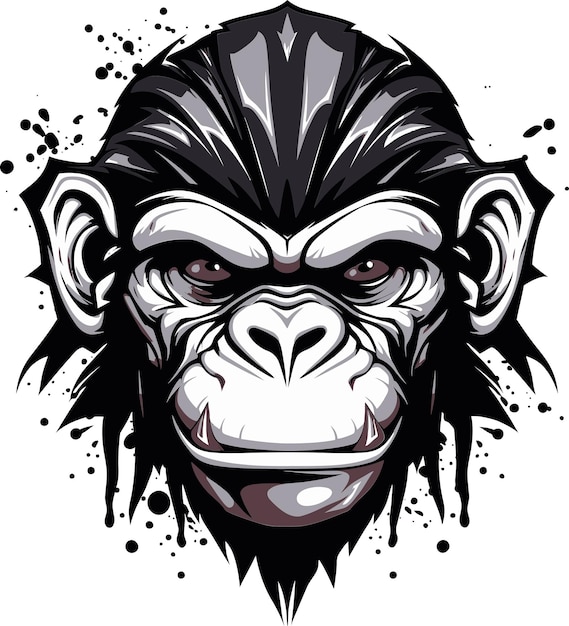The image depicts a menacing grayscale chimpanzee illustration rendered in black and white, set against a stark white background with ink splatter accents. The chimpanzee is facing forward, head-on, with dark, intense eyes that seem to have a hint of dark plum or red, adding a sinister touch to its expression. Its furrowed brows and sharp, prominent bottom canines enhance the intimidating look. The face is intricately detailed, highlighting pronounced wrinkles, ears, and deeply set eyes. The chimp's hair is slicked back, emphasizing its facial features that are dramatically shaded with strong shadows and highlights. The ink splatters around the image create a chaotic and artistic feel, suggesting a dynamic and expressive piece of artwork.